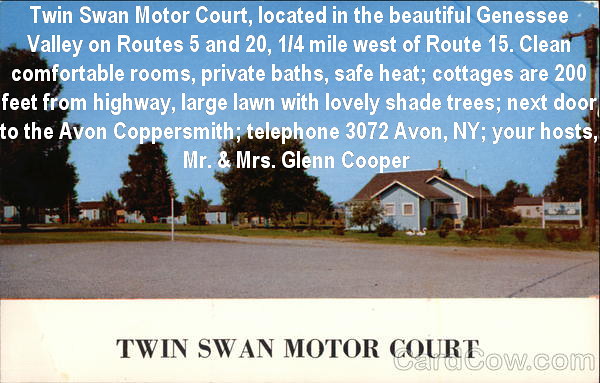The image is a detailed advertisement for the Twin Swan Motor Court, located in the picturesque Genesee Valley at routes 5 and 20, approximately one quarter of a mile west of route 15. The image showcases a serene neighborhood with a prominent house featuring gray rooftops and surrounded by lush green lawns and trees. A broad street runs in front of the house, accompanied by a walk path winding through the neighborhood. Adjacent buildings and more houses are visible in the background amid the green scenery.

Prominently displayed in white letters across the sky portion of the image is the promotion for Twin Swan Motor Court, highlighting its amenities such as clean, comfortable rooms, private baths, and safe heat. Notably, the cottages are set 200 feet away from the highway, offering a large lawn with lovely shade trees and proximity to the Avon Coppersmith. Essential information is provided, including the phone number (3072 Avon, New York) and the welcoming hosts, Mr. and Mrs. Glenn Cooper.

Beneath the photograph, on a white background, "Twin Swan Motor Court" is printed in bold black letters, and the ad includes the website "cardcal.com" in outlined gray letters. The image collectively serves as an inviting call to book a stay at this well-advertised motor court.